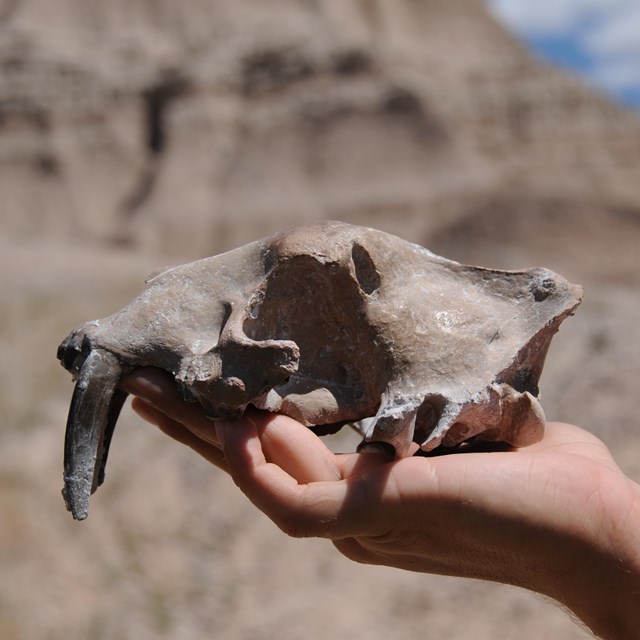In this detailed photograph, a white Caucasian person's left hand holds a fossilized skull, likely of a saber-toothed tiger, characterized by its distinct two long, saber-like teeth jutting downward. The background of the image is intentionally blurred, revealing hints of a desert-like, sandy ground that transitions into a rugged mountainside. Additionally, a blue sky with white clouds is partially visible in the top right corner, possibly indicating a vast, outdoor scene such as a mountainous region or an archeological dig site. The skull shows signs of degradation with one tooth more intact than the other, suggesting it has undergone fossilization over many ages.